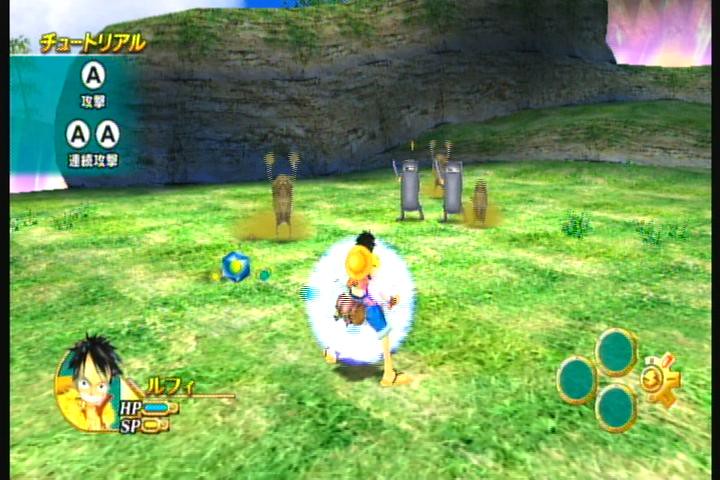The image is a screenshot from an 80s-style video game, likely Chinese due to the non-English characters at the top. The setting appears to be an outdoor area with a vast expanse of grass in varying shades, some patches looking sun-bleached. Dominating the background is a massive, mountainous rock formation capped with greenery. In the gameplay area, there are several medieval-styled characters with their hands raised. The focus is on a character donning a yellow hat, who seems to be emitting a powerful light, possibly using a superpower. This character stands out with a white aura surrounded by blue jeans, and there's an intense flash that suggests an out-of-body experience or some special ability aimed at the medieval figures. On the upper left corner of the screen, there are Asian characters followed by white circles displaying the letter 'A', surrounded by black text, and an avatar in a yellow shirt labeled HP and SP can be seen. The right bottom corner features three turquoise circles and a gold symbol. The entire scene is vividly set on a green grass background, underlining the game's vibrant and detailed design.